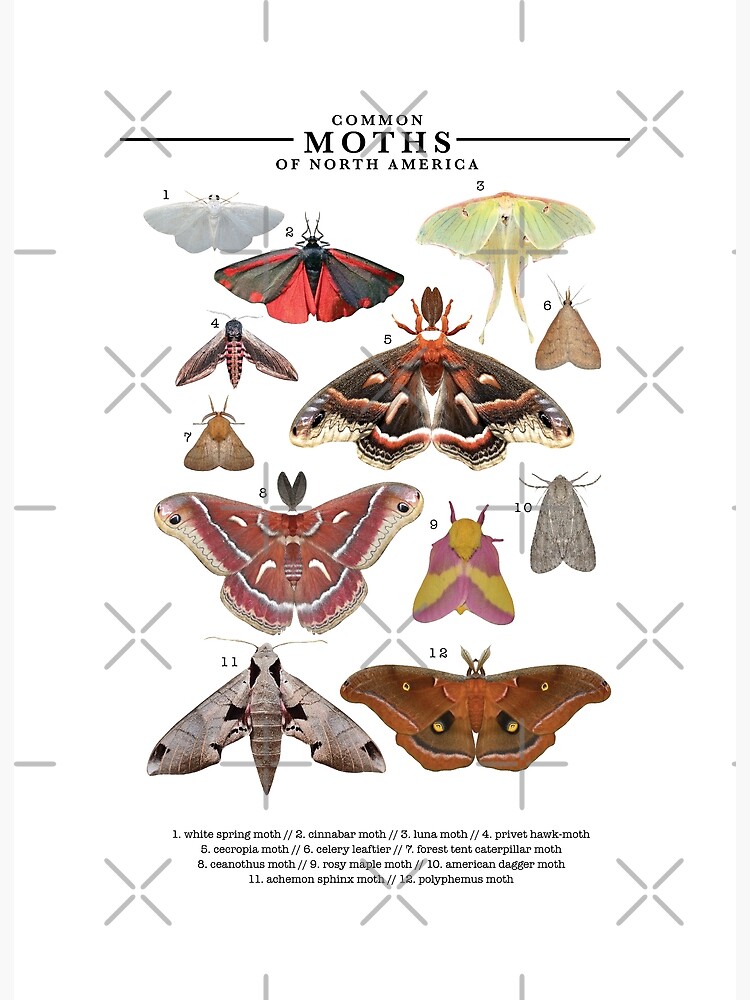The image is an educational poster titled "Common Moths of North America." It features 12 distinct moths, each photographed from above to showcase their diverse wing patterns and colors. The moths are numbered 1 through 12, corresponding to a legend at the bottom that identifies each one: 

1. White Spring Moth (white)
2. Cinnabar Moth (red and black)
3. Luna Moth (greenish-yellow)
4. Privet Hawk Moth
5. Cecropia Moth
6. Celery Looper
7. Forest Tent Caterpillar Moth
8. Ceanothus Silk Moth
9. Rosy Maple Moth (pink and yellow)
10. American Dagger Moth
11. Achemon Sphinx Moth
12. Polyphemus Moth.

The moths vary in size, from small to extra large, and display a wide array of colors including white, red, black, greenish-yellow, pink, yellow, brown, gray, beige, and reddish-brown. The page includes subtle gray X's, plus signs, and dashes as a background watermark, which do not distract from the clarity and detail of the moth photographs.